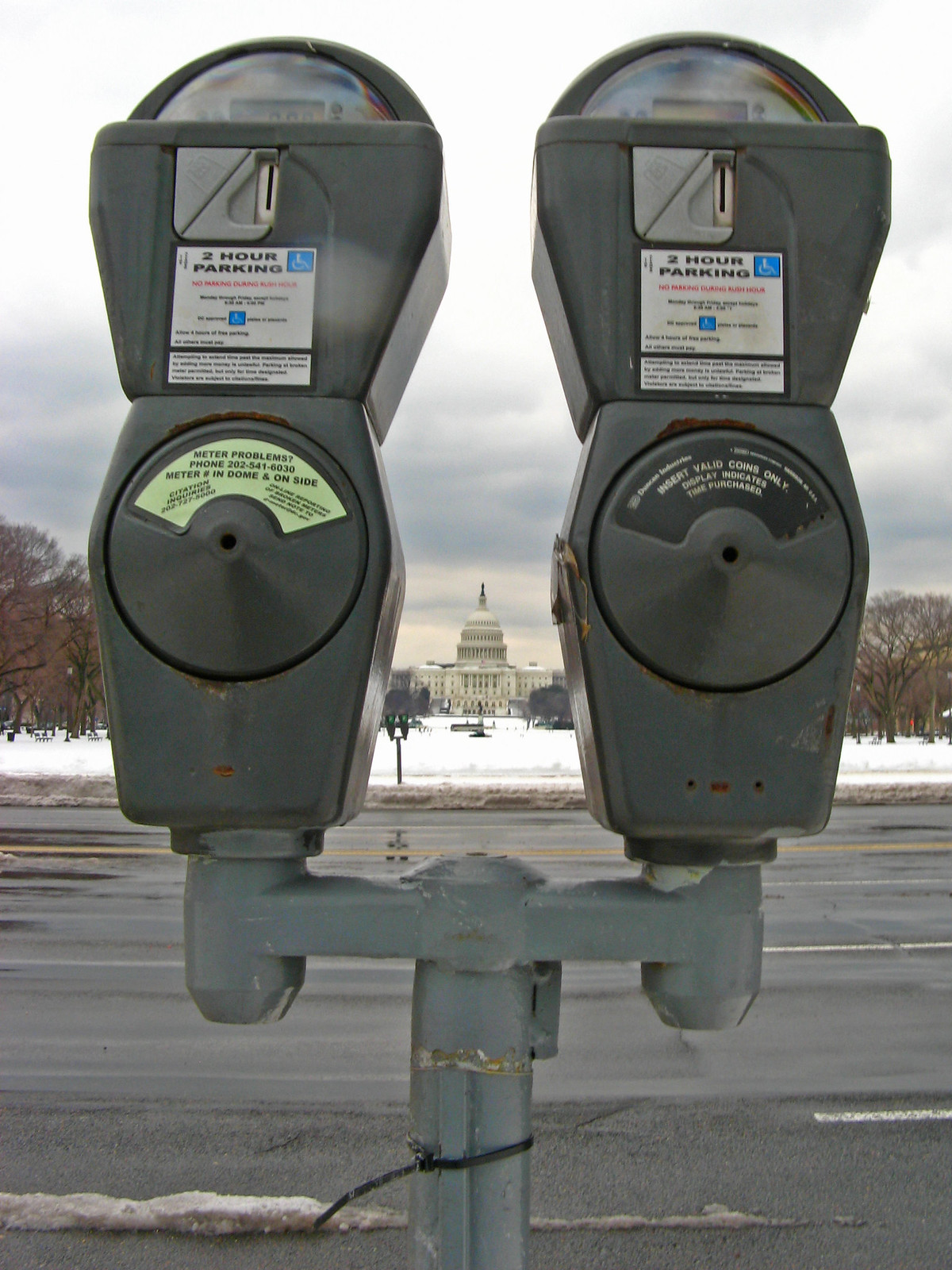The photograph captures a detailed close-up of a dual-style, gray-painted metal parking meter, set against the backdrop of a snowy, overcast winter scene. Each meter, mounted on a single post with two gray arms, features signage for two-hour parking, including a handicap symbol and information about meter problems with a contact number (202-541-6030). The photo is taken from a low angle, emphasizing the meters' presence. Between the two meters, the iconic U.S. Capitol Building is visible in the distant background, adding a significant landmark context to the urban setting. The ground is blanketed in snow, the roads are wet with slush, and the leafless trees accentuate the cold, wintry atmosphere. The sky above is gray and heavy with clouds, reinforcing the season's bleak ambiance.